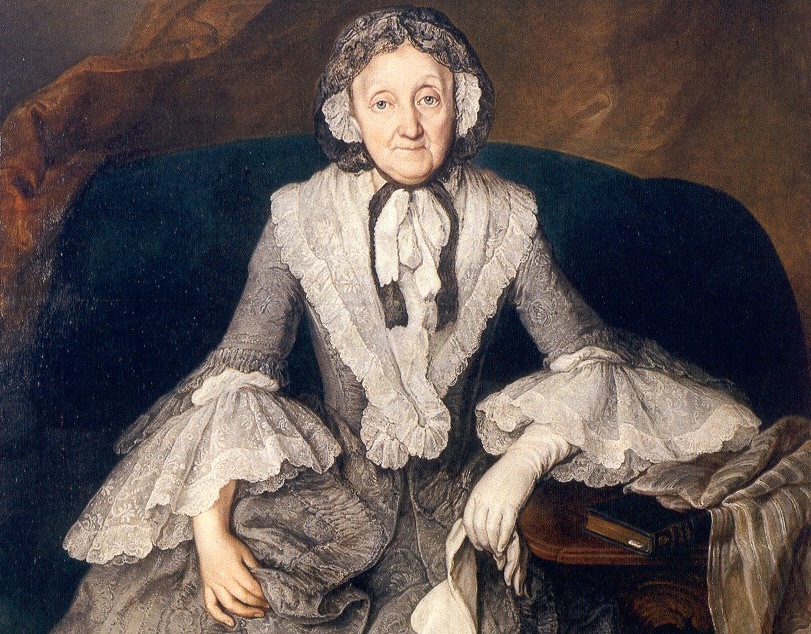This is a detailed and elegant portrait painting of an older woman, likely from the 1800s. The background is composed of rich brown tones, providing a stark contrast to her seated position in a luxurious, dark blue velvet chair. She appears to be in her seventies, characterized by her white hair adorned with a black, semi-transparent lace bonnet. Her blue eyes gaze forward, adding depth to her serene expression.

The woman is dressed in a light gray, old-fashioned Victorian dress that covers her from neck to toe. The dress is adorned with intricate white lace, especially noticeable on the crisscross lace around her shoulders and the flared flower-like lace cuffs at her elbows. One of her hands is adorned with a white leather glove extending up to her elbow, while the other glove rests elegantly in her lap.

Her arms are gently placed on a wooden table beside her, where a black book lies. The colors of the painting are a harmonious blend of grays, whites, browns, tans, and blues, creating a beautifully balanced composition. The painting does not reveal a visible signature, though there might be one subtly marked in the left-hand corner.